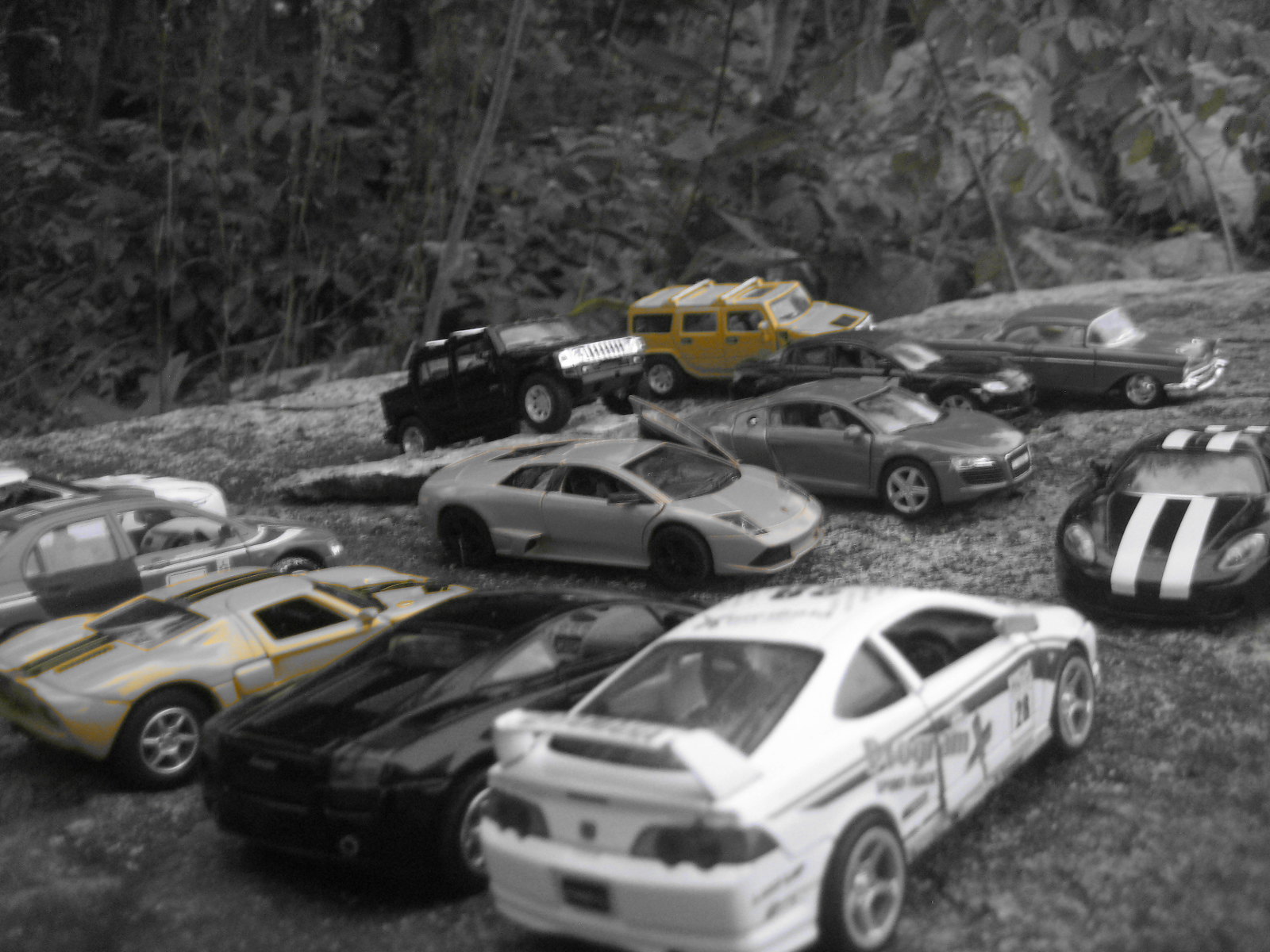The black and white photo, which appears to be slightly out of focus, captures an aerial view of a collection of cars parked on a grassy patch near a forest, creating a visually striking scene that almost resembles an elaborate model or toy car setup. The perspective and angle create an optical illusion, making it difficult to discern whether the cars are miniature models or real vehicles. The cars are meticulously detailed and arranged in a casual jumble. Closest to the viewer, there are five cars pointing away, and directly nose-to-nose with them is a black and white striped car facing towards the viewer. Among the various vehicles, which mostly seem to be luxury sports cars and off-road types, notable ones include a pale yellow Jeep-like vehicle and a pale gold car. Overall, there are ten cars in total, configured in various directions, including three cars in a perpendicular row and two more aligned behind them. The monochrome setting enhances the crisp, detailed look of the cars against the blurred, leafy backdrop of the forest.